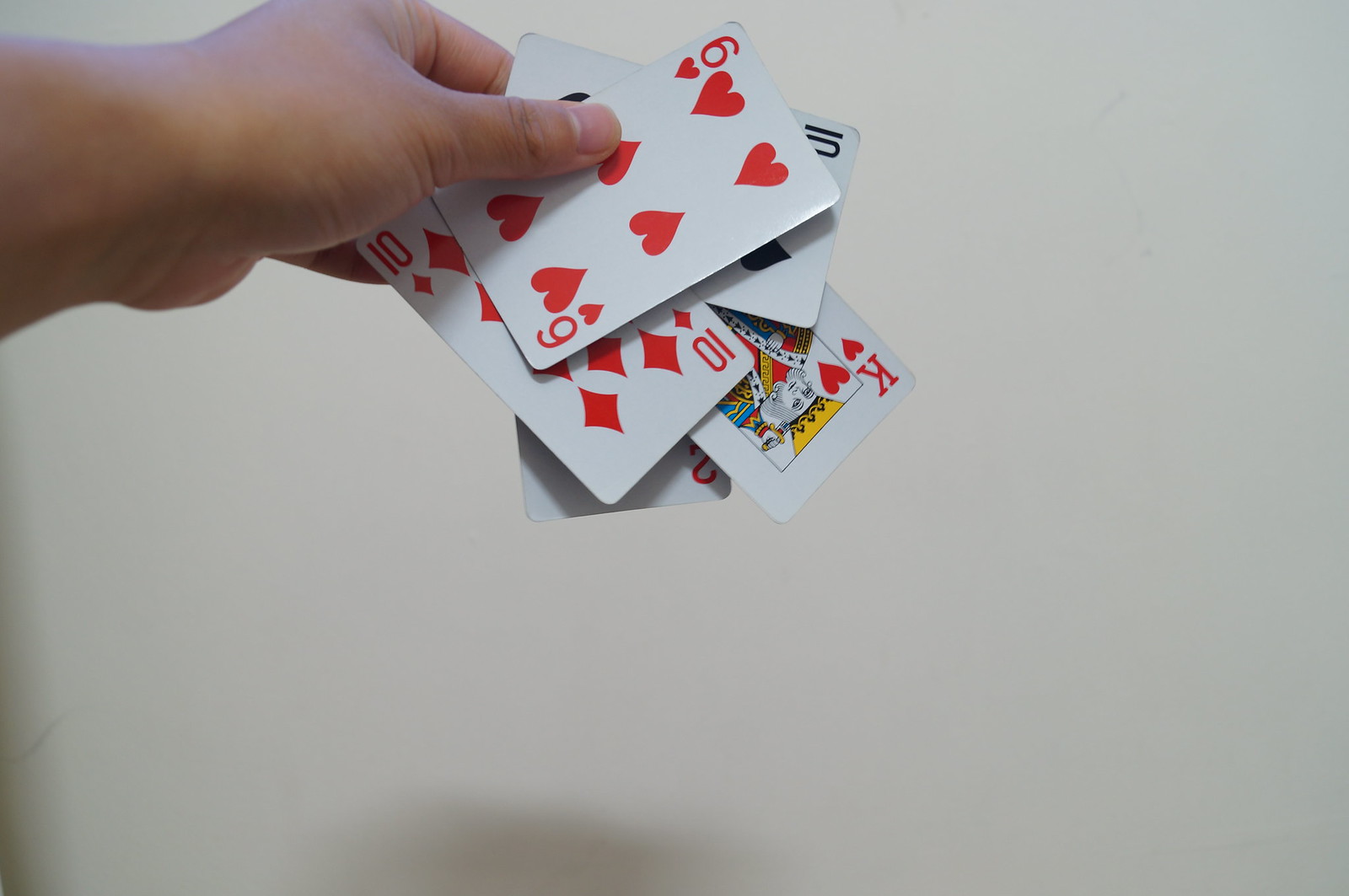In the image, a hand, possibly belonging to a Hispanic male, occupies the upper left corner of a rectangular background that should be white but appears gray. The hand, light tan in color, is holding five playing cards between the thumb and fingers. The cards displayed are: a six of hearts, with a white background and red heart symbols; a ten of spades, with a white background and black spade symbols; a ten of diamonds, with a white background and red diamond symbols; and a king of hearts, featuring a white background, red heart symbols, a gold crown, and intricate red, blue, and gold details. The fifth card is partially obscured, revealing only a '2' and leaving its suit uncertain, though it could be diamonds or hearts.